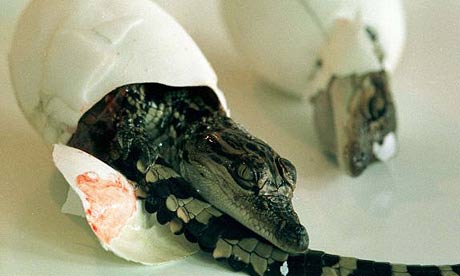The photograph features two hatching eggs placed on a hard white surface. Both eggs appear to be in the process of cracking open, revealing baby reptiles. The egg in the front left is in sharper focus and shows a baby crocodile emerging, with its head and tail protruding from the shell. Notably, there's a smear of blood on the left eggshell. The second egg, situated in the back right, is less focused, capturing only part of the eggshell and the reptile inside. The baby reptiles have black and light gray bodies, with some dark green and striped patterns visible. The setting suggests a controlled environment, possibly at a zoo or wildlife facility. The image is free of text, emphasizing the raw and natural detail of the hatching process.